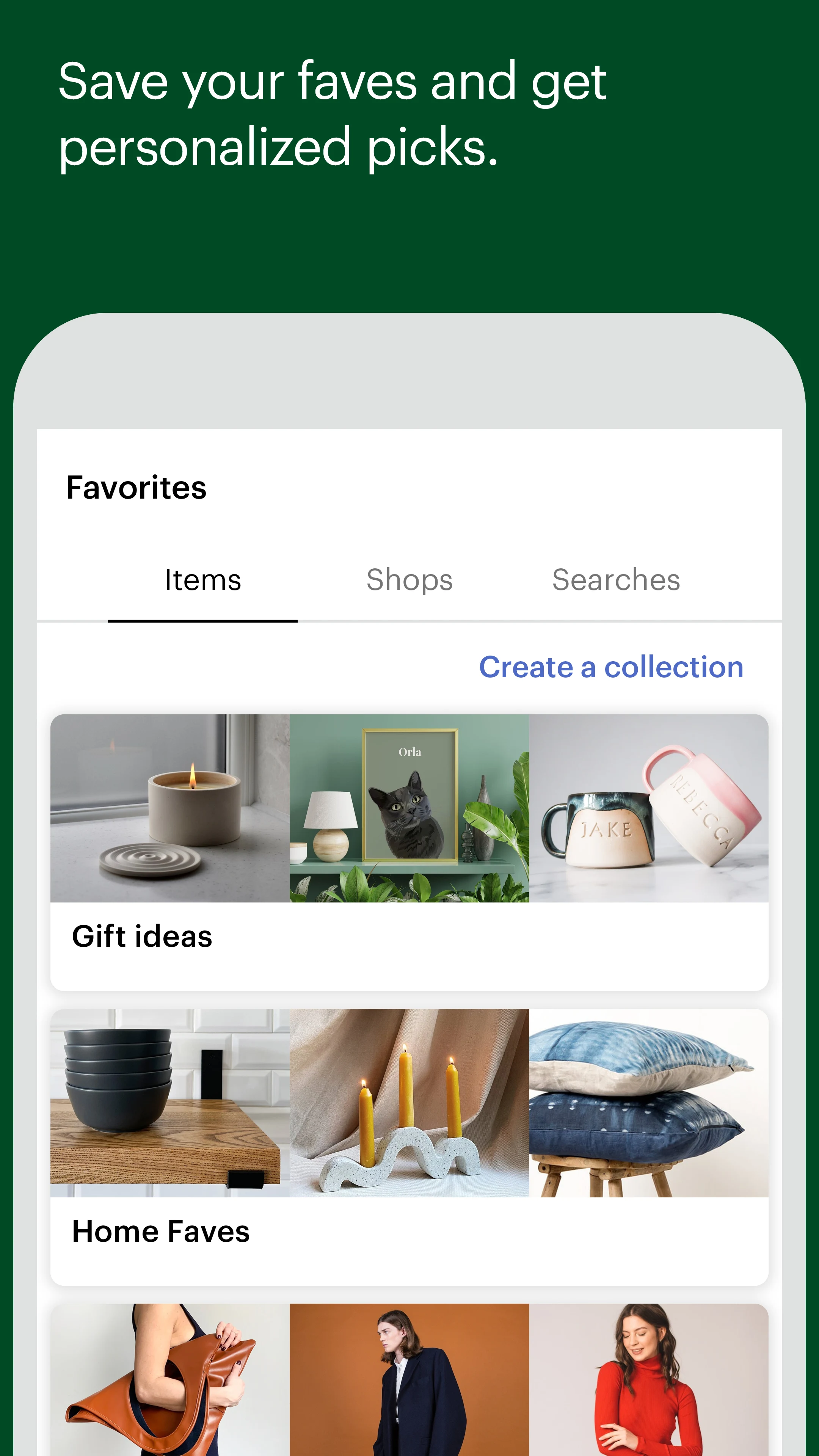This screen-capture image, taken from a mobile phone in portrait mode, displays an app or website interface against a rich, forest green background. Occupying the upper portion of this screen, white text reads, "Save your faves and get personalized picks.” 

Dominating the lower three-quarters of the screen is a prominent grey pop-up with rounded corners, within which lies a white rectangular section. At the top of this white section, the word "Favorites" is clearly marked in black text. Just below this label, there are three tabs: "Items," which is highlighted in black and underlined to indicate it is the current selection, followed by "Shops" and "Searches," which are greyed out.

Beneath these tabs is a vibrant blue button inscribed with the words "Create a Collection." 

The main content area features horizontally aligned rows of thumbnail photographs, categorized into different sections. The first row is titled "Gift Ideas," showcasing images of a candle, a framed picture of a cat, and some coffee mugs. The second row down, labeled "Home Faves," displays a stack of black bowls, a curvy candle holder, and two throw pillows atop a stool. 

The third row is partly cut off, leaving its title illegible, but the visible thumbnails depict items including a uniquely styled brown handbag, a dark blue pea coat, and a red turtleneck.